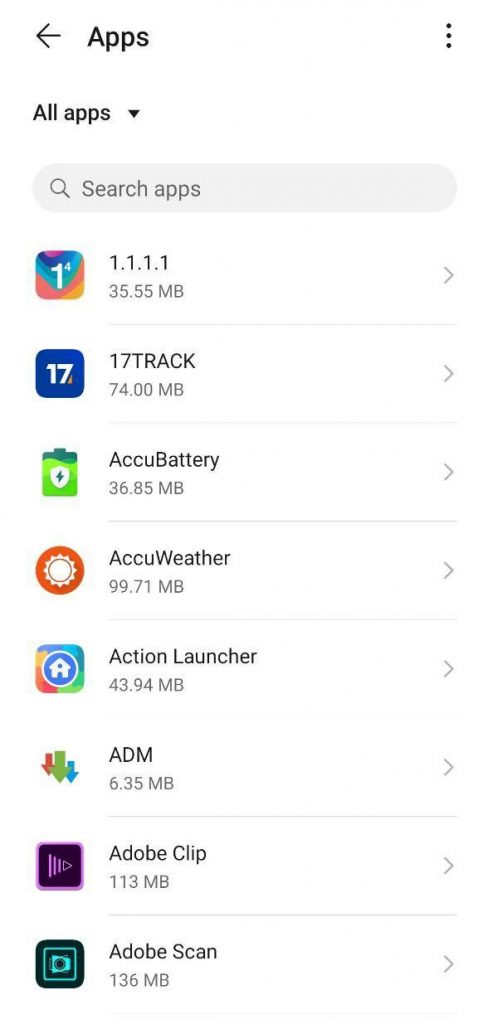In the top left corner, there's an arrow pointing to the left accompanied by the label "Apps". On the top right, there are three vertically aligned dots. Back on the left side, there's the label "All Apps" with a downward-facing arrow. Below this, there's a grey, rounded rectangle with a bulging shape at both ends, containing a magnifying glass icon and the text "Search Apps". 

Further down, there is a colorful square featuring the number "1" next to an indiscernible element. Adjacent to this, there is black text with a right-facing arrow. This section is divided by a grey line. 

Next, a blue square with the number "17" is present alongside some text and another right-facing arrow, followed by another grey dividing line. Below this, an icon resembling a battery, colored green and blue, sits next to some text and a right-facing arrow, with yet another grey line beneath it.

Following this, an orange circle with an image of the sun within it is placed next to some text and a right-facing arrow, underlined by a grey line. Then, there's a colorful square featuring a blue circle outlined in white with a white house inside it, accompanied by text and a right-facing arrow, with a faint grey line underneath. 

Below this section, three downward-facing arrows in orange, green, and blue are positioned next to text and a right-facing arrow, separated by a grey line. 

Next, a dark purple square outlined in lighter purple contains a triangle made of lines, followed by text and a right-facing arrow, underlined by another grey line. 

At the bottom, there's a dark blue-green square with a light blue element in the center, possibly containing a picture, with some accompanying text and a right-facing arrow.